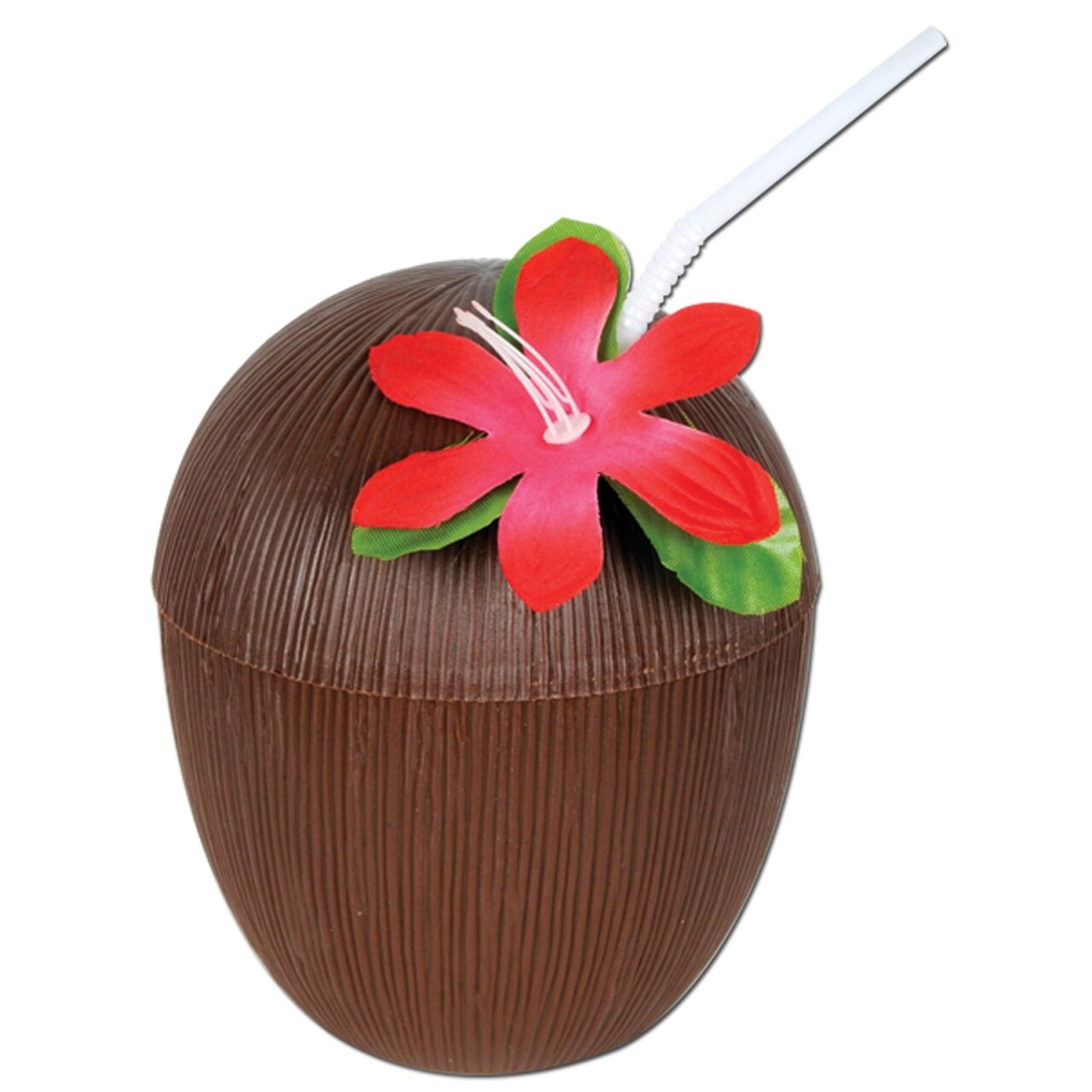This image depicts a 3D representation of a coconut-shaped cocktail cup, seemingly made from brown plastic with vertical ribbing but lacking the natural texture of a real coconut. The cup is topped with an intricately detailed artificial flower and leafy decoration. The flower, which is quite large, has six red petals with a white segment in the center from which white stringy filaments emanate, mimicking the appearance of natural flower stamens. Surrounding the flower are a few lifelike green leaves. A white flexible straw, featuring a faint gray or blue line, emerges near the floral arrangement. The background of the image is completely white, bringing sharp focus to the coconut-like cup and its vibrant decorative elements.